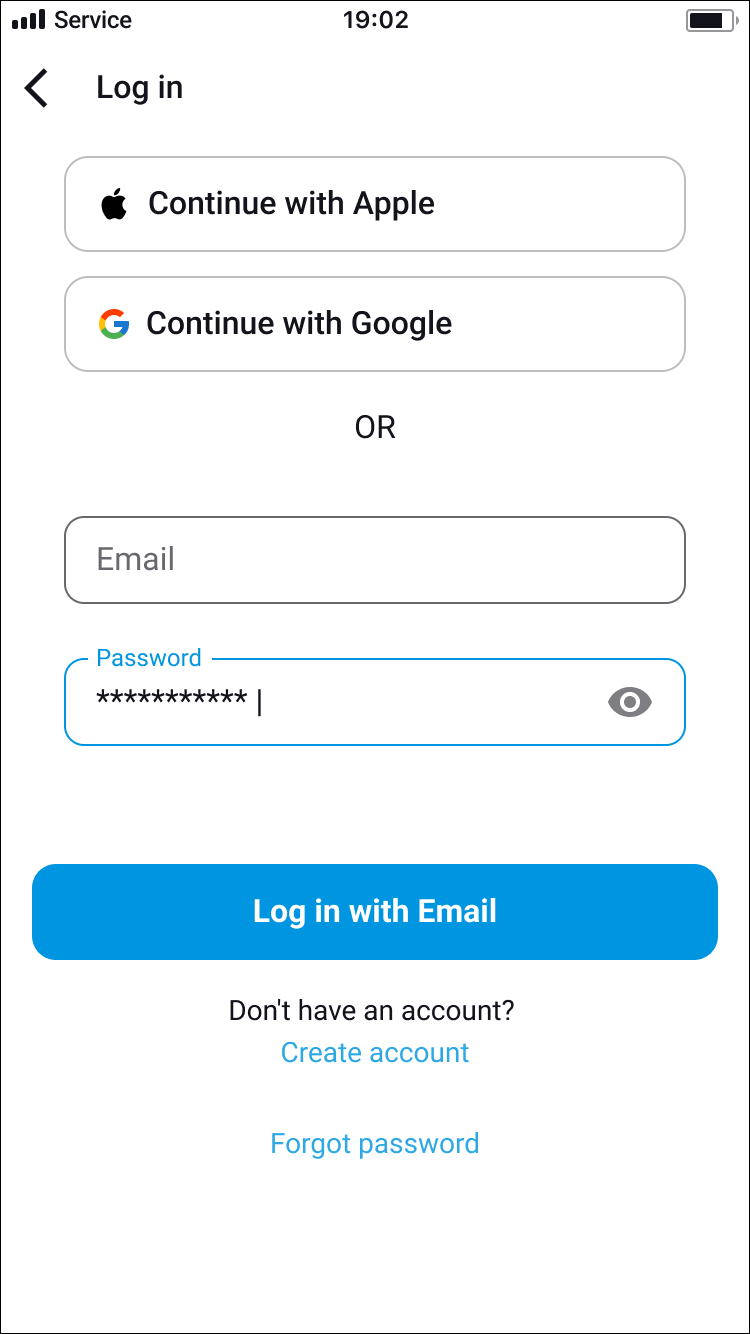The image displays a rectangular page with a white background that resembles a login screen for a digital application. At the very top of the page, there are four fully-filled bars indicating strong mobile service signal, followed by the word "Service." In the center at the top, the time is displayed as "19:02." On the top right corner, a battery icon shows a charge level of around 75-80%.

Just below this top section, the page features the heading "Login" accompanied by the Apple logo with the text "Continue with Apple," and directly below, the Google logo with the text "Continue with Google." Further down, the word "OR" separates these login options from the email login form.

The form includes two horizontal rectangular input boxes. The first box is labeled "Email," and the second box, labeled "Password," contains numerous asterisks (approximately 10 or 11) to obscure the entered password. To the far right within the password box, an eye symbol is present, likely indicating a function to show or hide the password.

Directly below these fields, there is a medium blue rectangular button with white text that reads "Login with Email." Beneath this button, in black text, it prompts users with the phrase "Don't have an account?" and, centered right below it in blue text, a "Create Account" link is available for new users.

A bit further down the page, still in blue text, the option "Forgot Password" is presented. The remaining lower portion of the page is blank, with no additional elements or text.